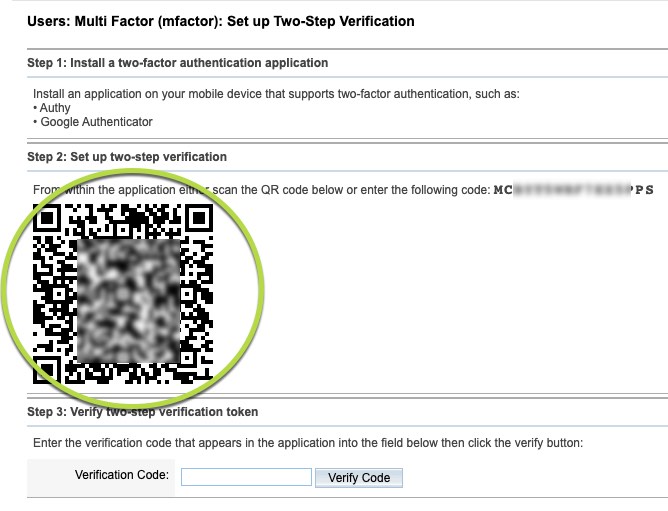This image is a screenshot depicting the steps to set up a two-factor authentication process, captured in landscape orientation with thin gray borders at the top and bottom. The image text includes the following details:

- **Header:** "Users, Multi-Factor, M-Factor, Setup, Two-Step Verification" (in black text)
- **Section 1:** 
  - Title: "Step One: Install a Two-Factor Authentication Application" (with a darker border on top and a lighter border on bottom)
  - Description: "Install an application on your mobile device that supports two-factor authentication, such as Authy or Google Authenticator."
- **Section 2:**
  - Title: "Step Two: Set Up Verification" (separated by narrow gray lines as borders)
  - Description: This section features a large white space with a prominently zoomed-in and highlighted QR code circled in green. The instructions beside it read, "From within the application, either scan the QR code below or enter the following code," followed by a partially redacted code for security.
- **Section 3:**
  - Title: "Step Three: Verify Two-Step Verification Token" (followed by a border below)
  - Description: "Enter the verification code that appears in the application into the field below, then click the verify button."
  - Additional Detail: Within a gray box with black font, it says "Verification Code," followed by a white input box with a blue border and another gray box labeled "Verification Code."

The image thus provides a comprehensive guide to setting up two-factor authentication, featuring clear instructions and protective measures for user security.